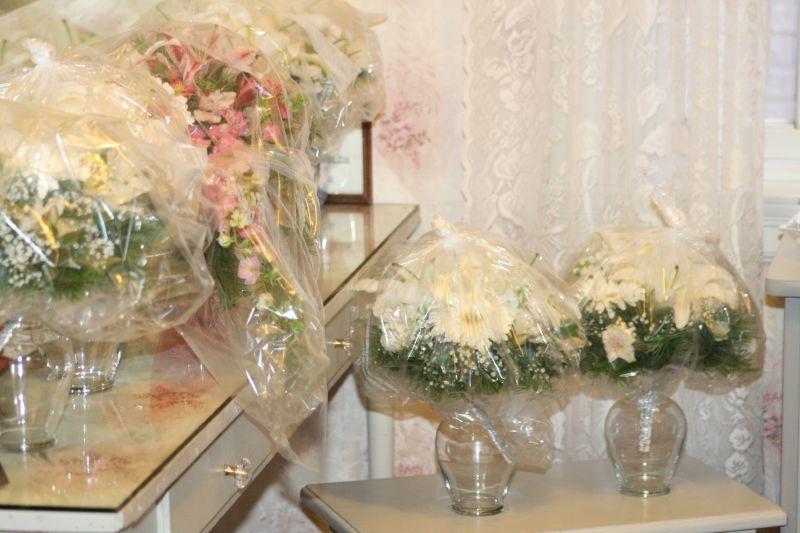The photo is an indoor, vintage-looking image with noticeable distortion or low-quality characteristics. The setting features a room with white lace curtains over a white-trimmed window. On the left side, there's a small, feminine desk with a pinky beige top and thin, pull-out drawers adorned with singular circular diamond designs. The desk, which has a marble-like light cream countertop and golden handles, hosts several clear vases filled with flowers. Most of these flowers are white with green leaves, although there are occasional pink and red ones. All flowers are covered in clear plastic bags.

Adjacent to the desk, there is an uncomfortable-looking white seating bench also topped with clear vases containing flowers. Additionally, there's a white table at the bottom right of the photo, which holds more vases. The room has white walls with a pattern and a brown-framed picture with a white background. The window, only partially visible, is dressed in white floral curtains that add to the quaint, nostalgic ambiance.